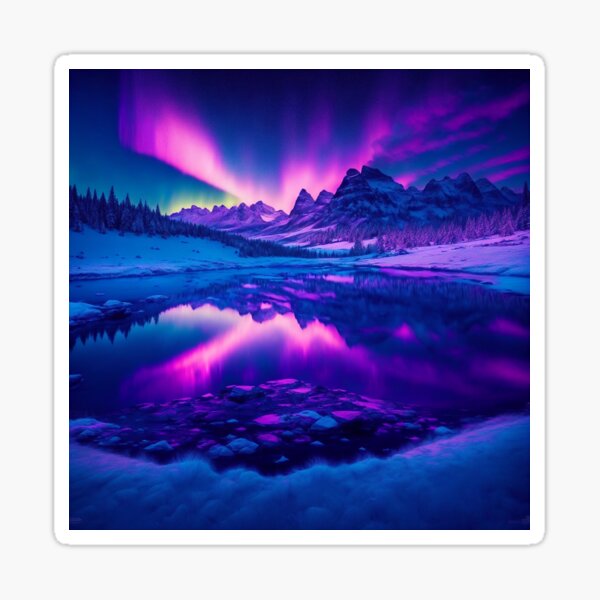This artwork is a rectangular painting with a border comprising a thin, rounded white outline followed by a thicker light gray border, set against a whitish-gray wall. The central scene showcases a mesmerizing winter night paradise dominated by hues of blue, pink, purple, and yellow. The sky is painted with a blend of these colors, featuring wavy and bright lights emanating behind a sprawling mountain range. The mountainous backdrop is tinted purple and white, indicating snowy peaks enhanced by the reflected purple sunlight.

In the foreground, to the left of the mountains, evergreen trees rise amidst a snow-covered ground, while similar smaller trees populate the right. The snow continues to blanket the terrain on both sides of the painting, leading towards the middle which contains a reflective body of water—a pond or lake. This water mirrors the vibrant sky and colors of the surrounding landscape. At the base of the painting, the shore is detailed with rocks that catch the blue and purple light from the sky above, seamlessly blending into the snow-covered ground that stretches from one side of the image to the other.